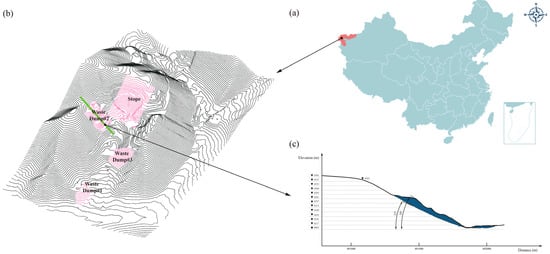The image is a detailed digital diagram featuring two maps and a graph, illustrating a geographic and topographic study. In the top right corner, labeled with a lowercase "a" in parentheses, there is a map which appears to depict a region that may be part of the former Soviet Union. This map, predominately teal with white boundary lines and a compass pointing north, includes a highlighted red section in the top left area. An arrow from this map points to "B," which shows a 3D representation of the terrain, enlarging and detailing the red-highlighted area from "A." This second section, though blurry, displays gray hill-like structures with pink-highlighted parts and another arrow pointing to "C." The final part, labeled "C," is a line graph that slopes from left to right, featuring dark teal markings along the slope. The graph is too small to read specifics, but it completes the study by visually connecting the geographical data with numerical analysis. The overall color scheme incorporates light blue, gray, pink, and dark blue elements, emphasizing the detailed and layered nature of the study.